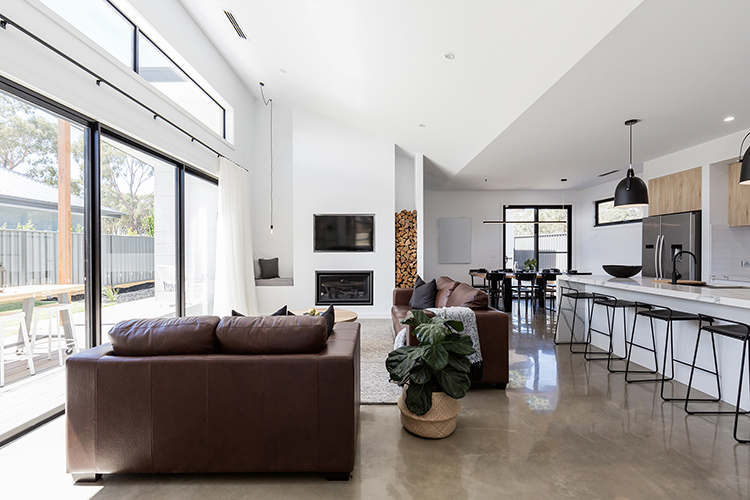The image is a horizontally aligned rectangular picture taken inside a modern house with an open floor plan, featuring brown tiled flooring and white walls and ceilings. On the left side, there are three large floor-to-ceiling windows with black trim, which allow a view of an exterior fence, a picnic table under a covered porch, another house, and trees in the background. Below these windows, an area with drapery is visible next to a green plant in a beige pot.

Inside, on the lower left corner, there's a dark chocolate leather love seat facing the windows and a brown leather sofa placed perpendicular to it, creating a cozy seating area. A TV is mounted on the wall with a built-in fireplace below it. To the right of this setup, there is a cut-out in the wall containing a stack of firewood. 

On the right side of the room, a long white marble countertop with a black bowl on top extends from the center right towards the center of the image. Five to six black, flat-topped barstools with metal legs, without backs, are lined next to the counter. Above the counter, two black pendant lights hang from the ceiling. Adjacent to the countertop, a dark silver refrigerator is visible along with light brown cabinetry.

Towards the far end of the room, a single glass door or large glass window stretches from the floor almost to the ceiling, accompanied by a round kitchen table with black chairs. The kitchen area also features a sink with a J-shaped black handle. The overall design and layout of the room emphasize its modern and spacious aesthetic.